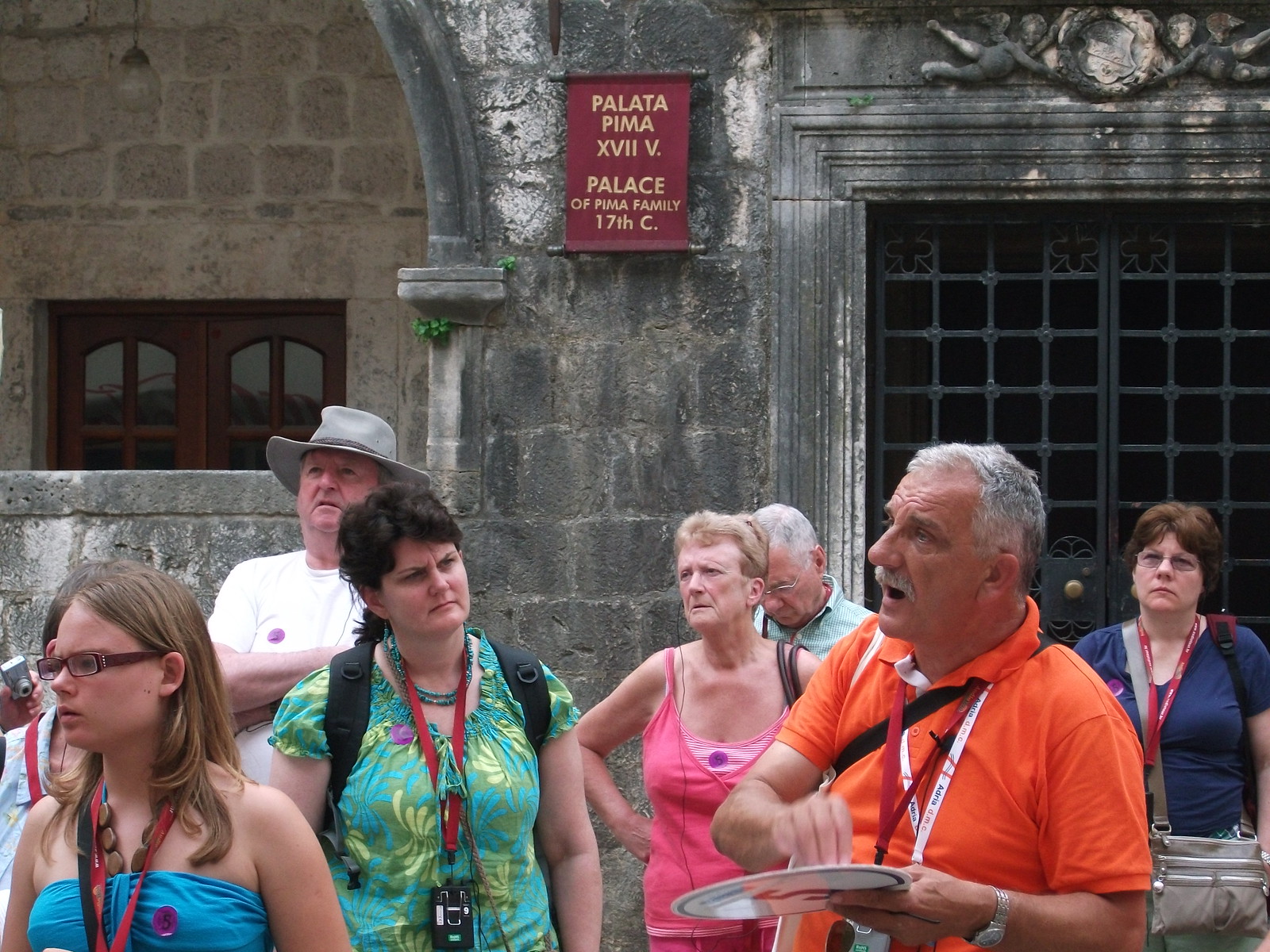In the photograph, a group of tourists is gathered outside an old gray stone building, identified by a burgundy and gold banner that reads "Palata Pima XVIIV, Palace of Pima Family, 17th Century." In the foreground stands the tour guide, an older man with short gray hair and a mustache, wearing an orange polo shirt and holding a sign with the number five. His mouth is open as if he's explaining something, pointing towards the ornate metal grate door on the right-hand side. The diverse group of tourists, comprised mostly of older adults and a few younger individuals, wear lanyards with identification cards around their necks. Among them is a woman with short brown hair in a multicolored shirt, another in a blue tube top, and an older lady in a pink tank top. They stand before the historical edifice, some looking at the tour guide and others gazing around, immersed in the experience.